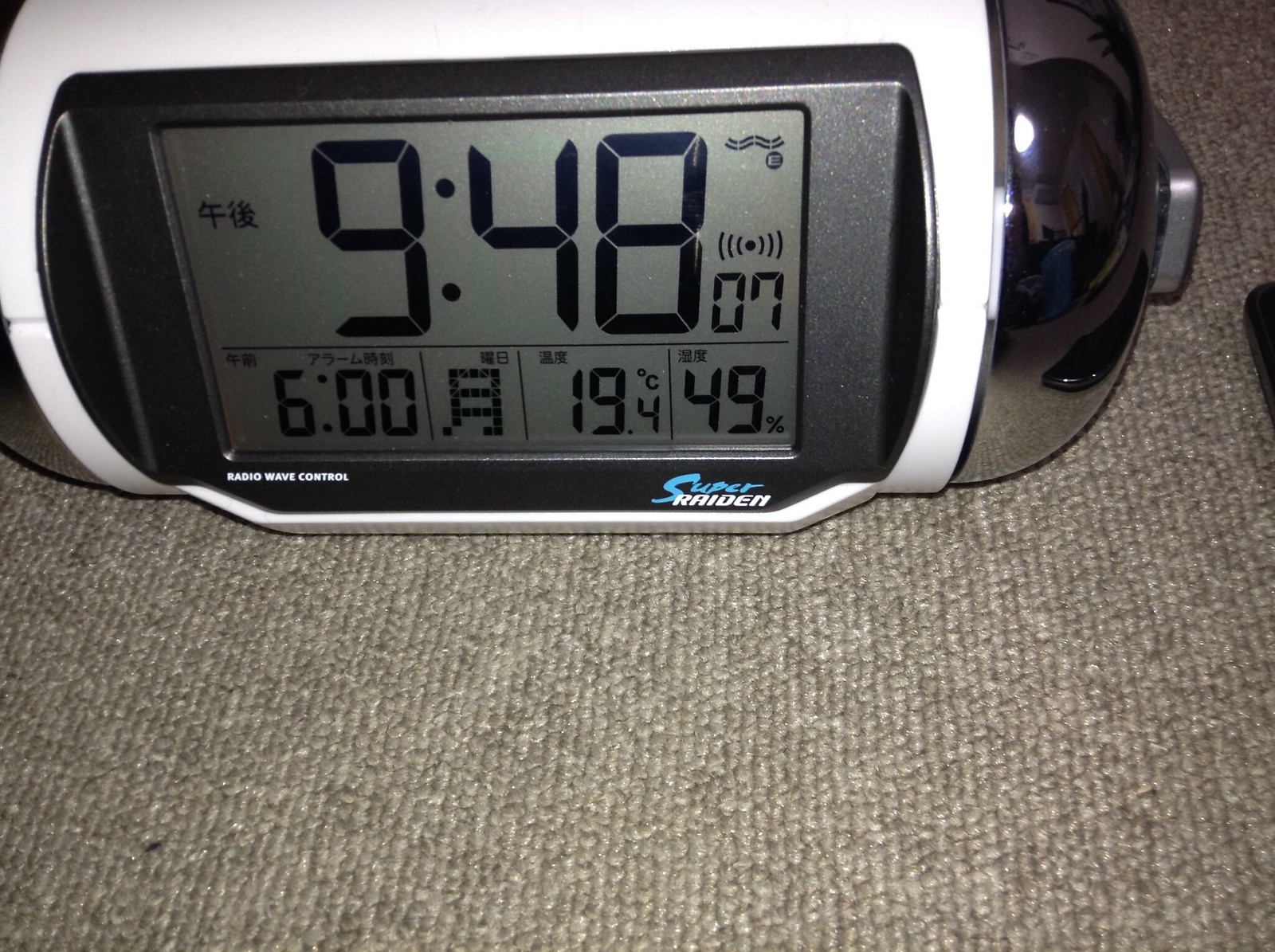This close-up photograph showcases a digital alarm clock, prominently placed on a gray Berber carpet with short nap. The clock features a unique design with a cylindrical shape and a front rectangular digital display panel. The housing of the clock is predominantly white with black accents around the display and shiny, reflective chrome on the ends. Additionally, there appears to be a handle pushed back behind the clock.

The digital display on the clock shows multiple readings: at the top, the time is displayed as 9:48:07, with Asian characters present above and around the numbers. Below this primary display, there are segmented sections. One section shows a secondary time at 6:00, another displays the temperature as 19.4 degrees Celsius, and a third section indicates a 49% reading, likely humidity. The bottom left of the display features the text "Radio Wave Control" in white, while the bottom right shows "Super Raiden," with "Super" displayed in sky blue and "Raiden" in white.